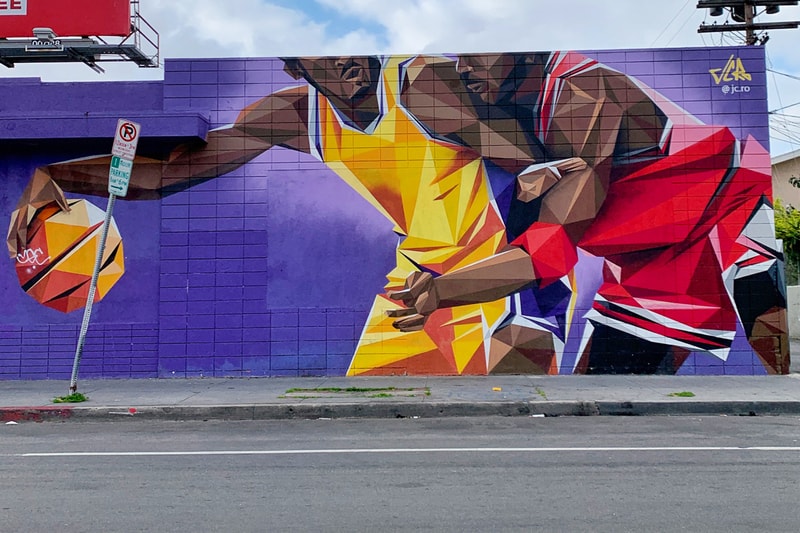This detailed photograph captures a vibrant outdoor mural painted on the side of a purple brick building, situated in an urban environment. The background features a light blue sky with numerous clouds. To the right, there is a brown house partially visible along with electric wires and a pole above the building. 

The mural itself predominantly showcases two African-American basketball players in mid-action. The player on the left, donning a yellow uniform trimmed in purple, is holding an orange octagonal basketball in his outstretched right hand. The opponent behind him is dressed in a red jersey trimmed with white and black, wearing a red wristband on his left arm. Both players' faces are only partially visible, cropped from the nose down.

Foreground details include a well-worn gray sidewalk with grassy patches, a bent "No Parking" sign, and a street marked by a white line. There is also a small orange sticker on the curb and some visible trash near a drain. A bit of another billboard with possible orange color is peeking from the top left, supported by scaffolding, and some discernible text including perhaps "VCR incorporated" and "@JCRO" is present on the mural. Noteworthy is the mural’s dynamic and geometric composition, blending elements of cubist style with bold colors such as red, yellow, orange, blue, purple, brown, black, and white. It artistically commemorates the figures, likely drawing inspiration from iconic players like Kobe Bryant and Michael Jordan, giving the scene a layered and soulful athletic spirit.